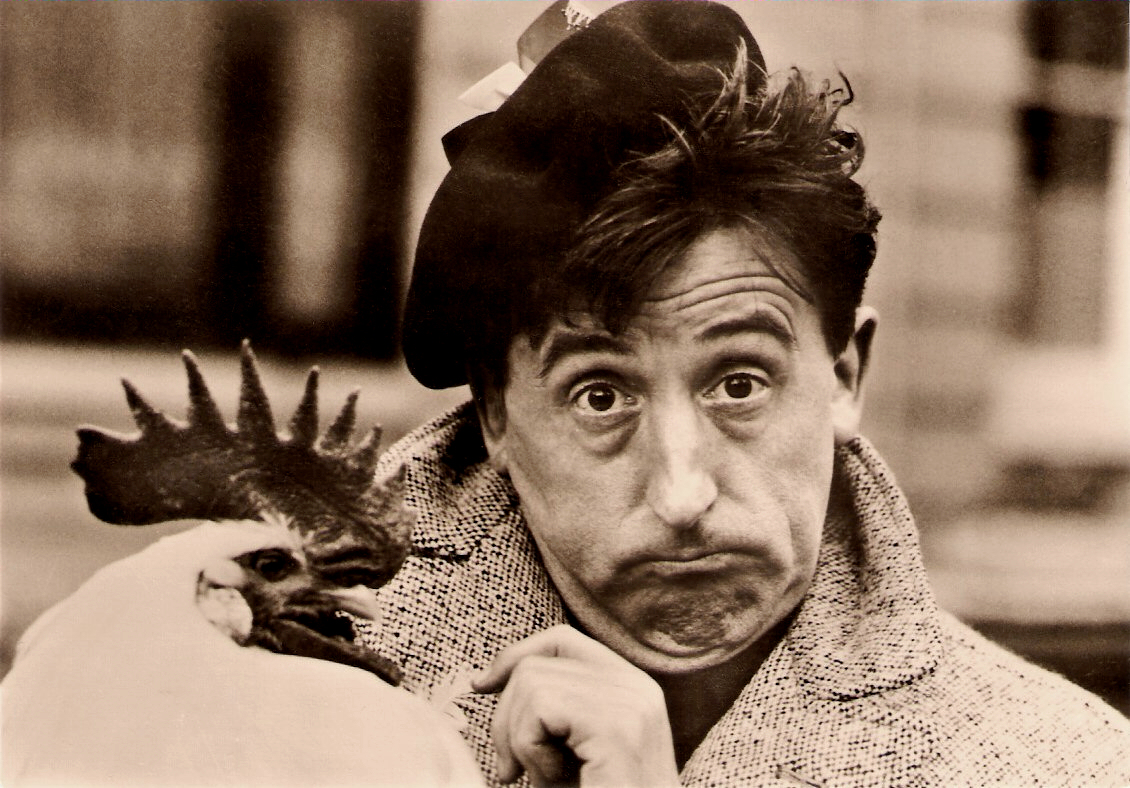In this black and white image, a man is wearing a dark beret, slightly tilted to the side, with strands of his dark, somewhat spiked hair peeking out from underneath. He sports a coat that may have a patterned texture and has his left hand raised, just beneath his double chin, which is dimpled and drawn back, giving his face a look of quizzical surprise. His wide-open eyes and raised eyebrows add to his humorous expression. 

On his left shoulder, a rooster is perched, partly cut off but clearly visible. The rooster’s comb appears dark due to the image’s monochromatic tone. The blurred background suggests an outdoor setting, though the focus remains sharply on the man and the rooster. The contrasting patterns and textures, combined with the man’s peculiar expression and posture, create a striking and somewhat comical scene.